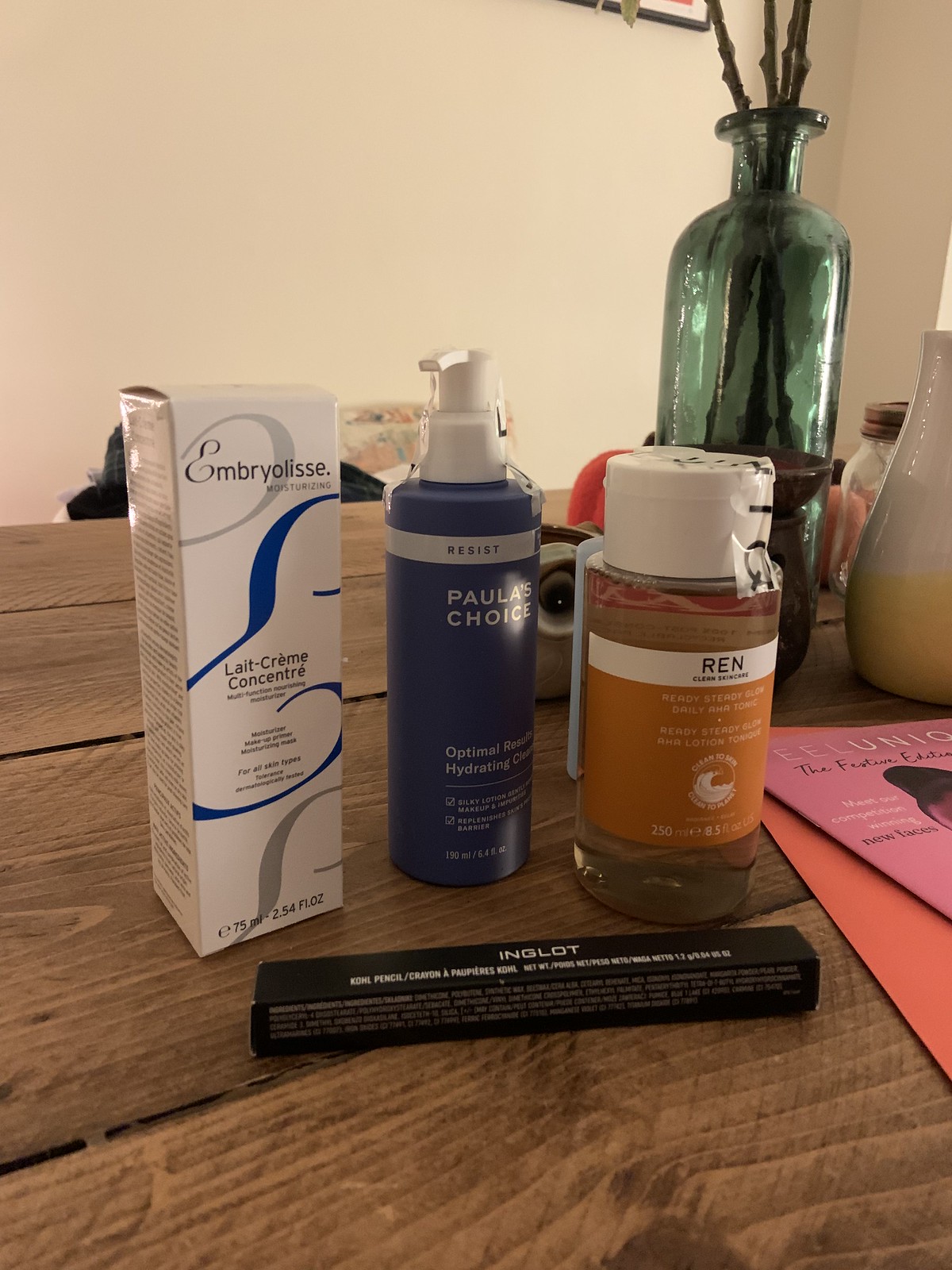A beautifully composed photograph showcases a collection of skincare essentials meticulously arranged on a wooden table. In the foreground, a sleek, long, thin rectangular box in black, emblazoned with the brand name "Inglot" in white letters, contains a kohl pencil for eye lining. Behind it, three distinct items stand in a neat row. 

On the left, a tall, rectangular white box from "Embryolisse" presents a multifunction nourishing moisturizer suitable for all skin types. Adjacent to it, a blue plastic bottle with a white pump from "Paula's Choice" reads "Optimal Results Hydrating Cream." Completing the trio, a clear bottle from "REN Clean Skincare," showcasing "Ready, Steady, Glow Daily AHA Tonic," boasts a large white, flip-top lid. Both the tonic and the hydrating cream are secured with tape, indicating they are freshly purchased.

To the far right, resting on the wooden surface, are two pamphlets. The bottom one is in a pale orange or peach hue, topped by a medium pink pamphlet. The pink one is titled "EELUNIO: The Festive," featuring a photograph of a woman on its cover. The entire scene is a testament to thoughtful curation, ideal for a skincare enthusiast.